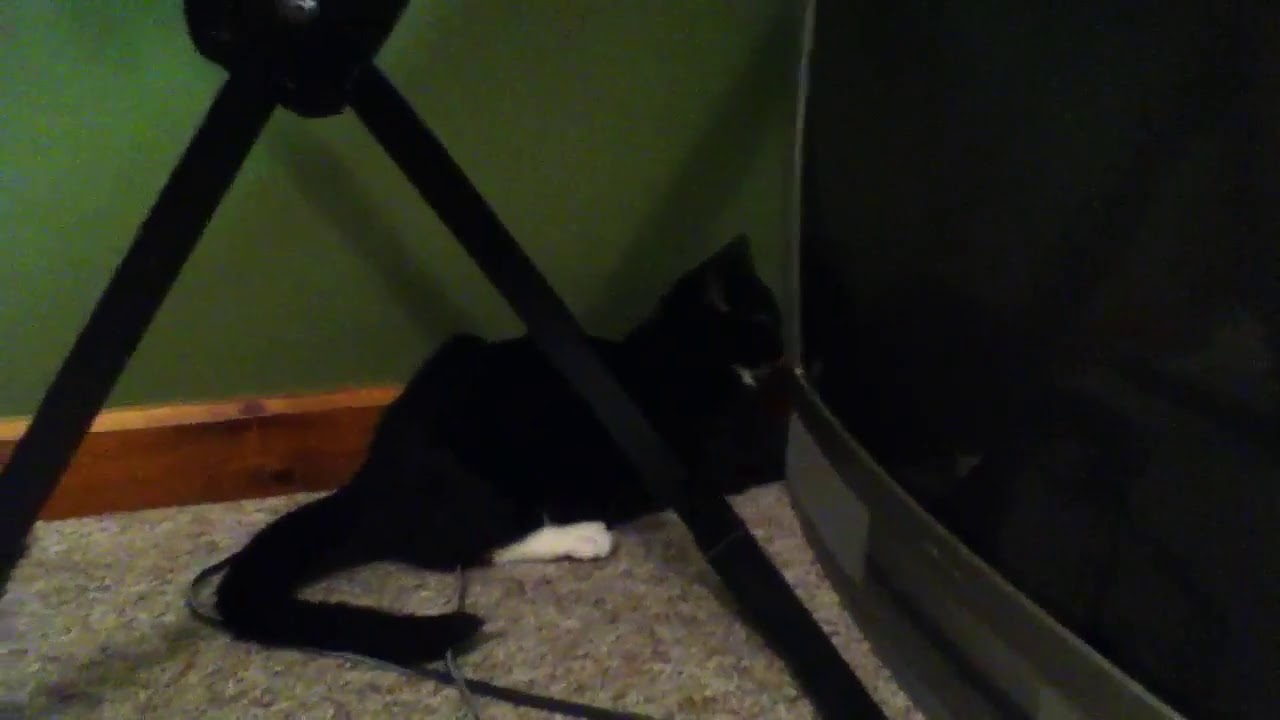In the image, a black cat with a partially white hind leg and white chest is laying on a tan carpet with brown and yellow tinges, along with some hints of gray. The cat appears to be playing or reaching into a small crevice between a thick, older model television on the floor and a green wall with a reddish-orange wooden trim at the bottom. Notably, the cat's tail is all black, and a cord runs underneath it. Above the cat, part of a stand with a V-shaped or X-shaped base is visible. The television has a black screen that's off and is framed by silver or gray. The cat's pose suggests it's intrigued by something behind or in the crevice next to the TV.